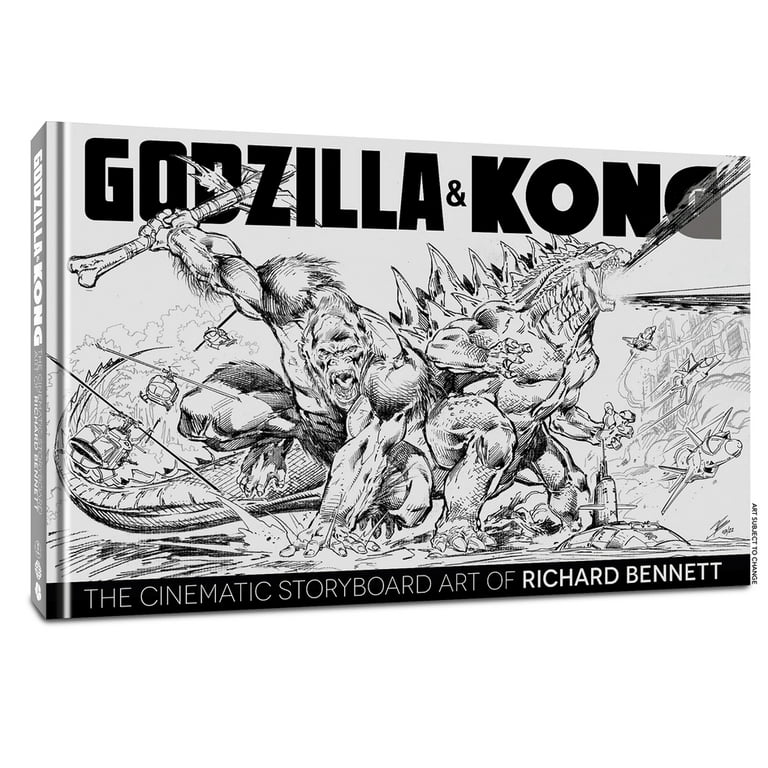This image depicts the cover of a graphic novel or book titled "Godzilla and Kong," emblazoned in large black letters against a light gray background at the top. The main artwork, rendered in black and white, showcases an intense scene: Kong, a massive gorilla, prominently occupies the left side with his mouth agape, one arm outstretched and the other gripping an axe with a bone handle. Behind and slightly to the right, Godzilla, the iconic dinosaur-like creature with pronounced spiky back ridges, is shown roaring, seemingly emitting energy from his mouth. Surrounding the two titans are various aircraft, including planes and helicopters, with additional details such as a jet engine-powered aircraft and a submarine near Godzilla. At the bottom of the cover, a black band features the white text, "The Cinematic Storyboard Art of Richard Bennett," identifying the artist behind the depiction. The book’s thick spine runs vertically along the left edge, also bearing the title "Godzilla and Kong" along with the descriptive text. In the lower right corner, small print notes that the "art is subject to change." The cover is set against a white background.